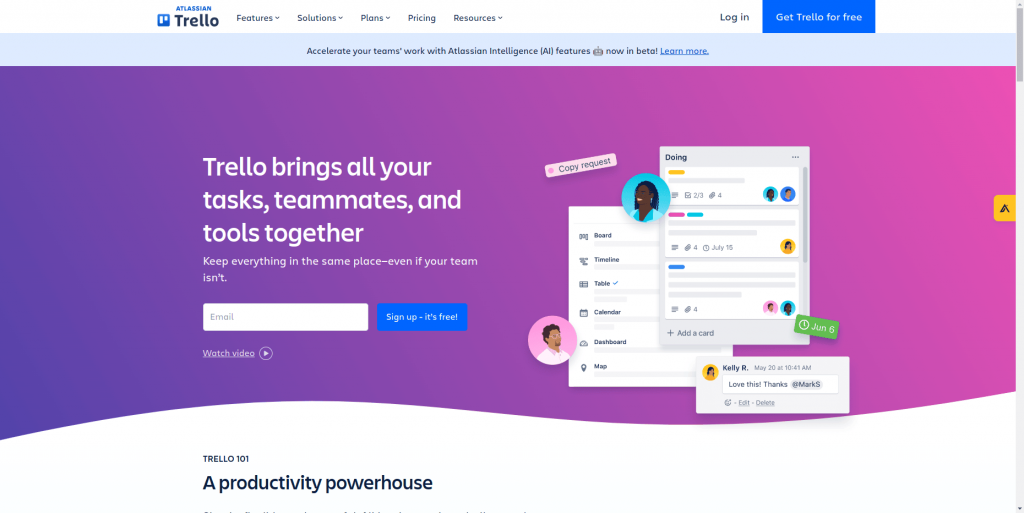Screenshot of Trello Homepage

The image captures the homepage of the Trello website. Prominently displayed on the upper left-hand side is the Trello logo. Adjacent to this logo is a menu bar containing several options: "Features," "Solutions," "Pricing," and "Resources." Each of these menu items includes drop-down options for further navigation. To the right on the same menu bar, there is a "Login" button followed by a "Get Trello for free" button, which is highlighted in a blue square.

Directly below the menu bar, there is a prominent section promoting the website's capabilities. The headline reads, "Accelerate your teamwork with intelligent AI features now in beta." Beneath this, another line states, "Trello brings all your tasks, teammates, and tools together. Keep everything in the same place even if your team isn’t."

At the bottom of this promotional section, there is an input text box where users can enter their email address to sign up for Trello’s services.